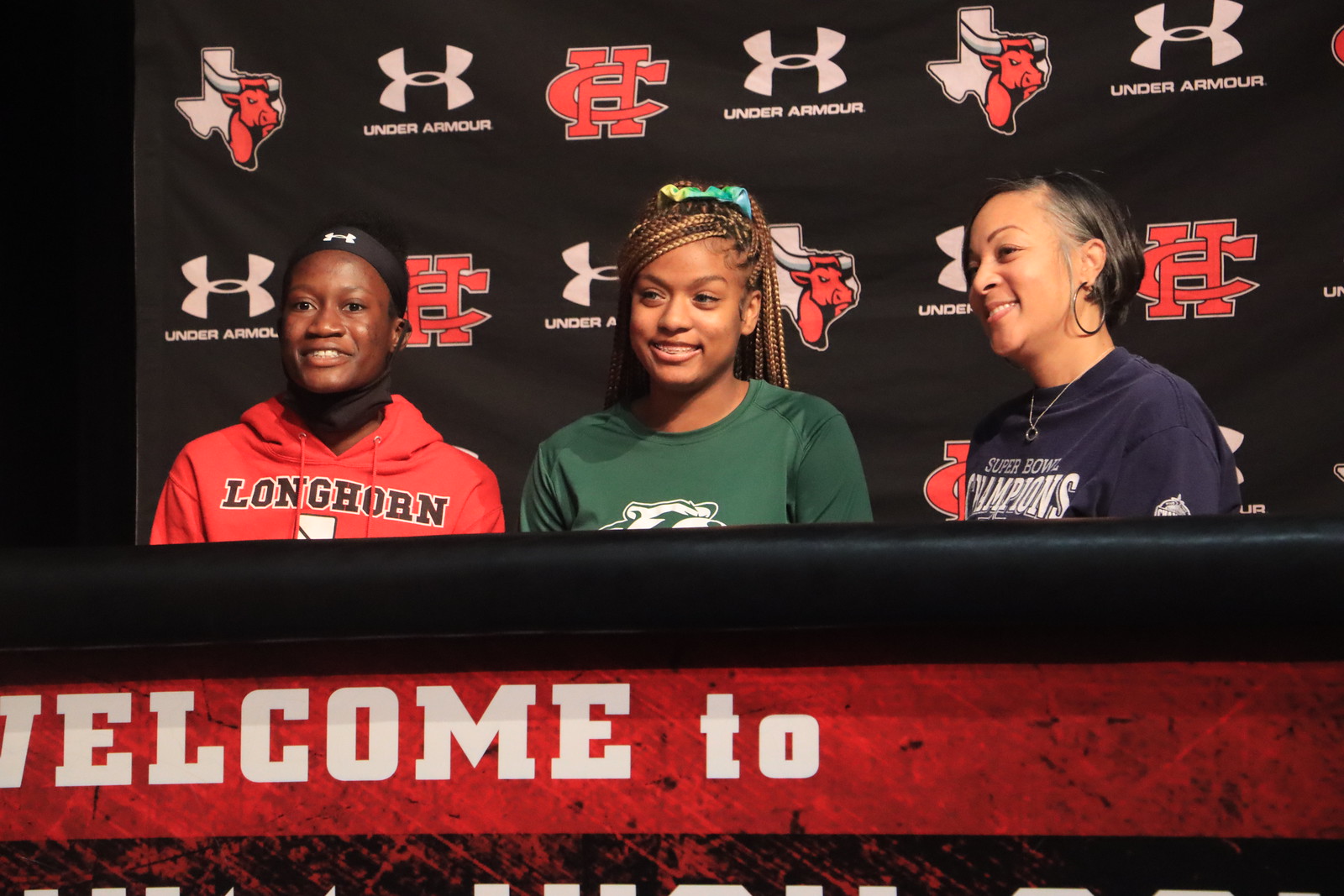The image depicts a scene resembling a press conference, featuring three African-American individuals seated behind a ledge. To the left is a young male in a red hoodie with "Longhorn" emblazoned on it, wearing a black face mask. In the middle sits a teenage girl, approximately 13-16 years old, dressed in a green shirt adorned with an animal emblem. To the right is a middle-aged woman, possibly in her 40s, sporting a navy blue "Super Bowl Champions" shirt. They are all smiling and looking towards the left side of the camera. The backdrop is black, prominently displaying logos including Under Armour, a bull inside a Texas map, and a “CH” emblem. A partially visible sign in front of them reads "Welcome to..."